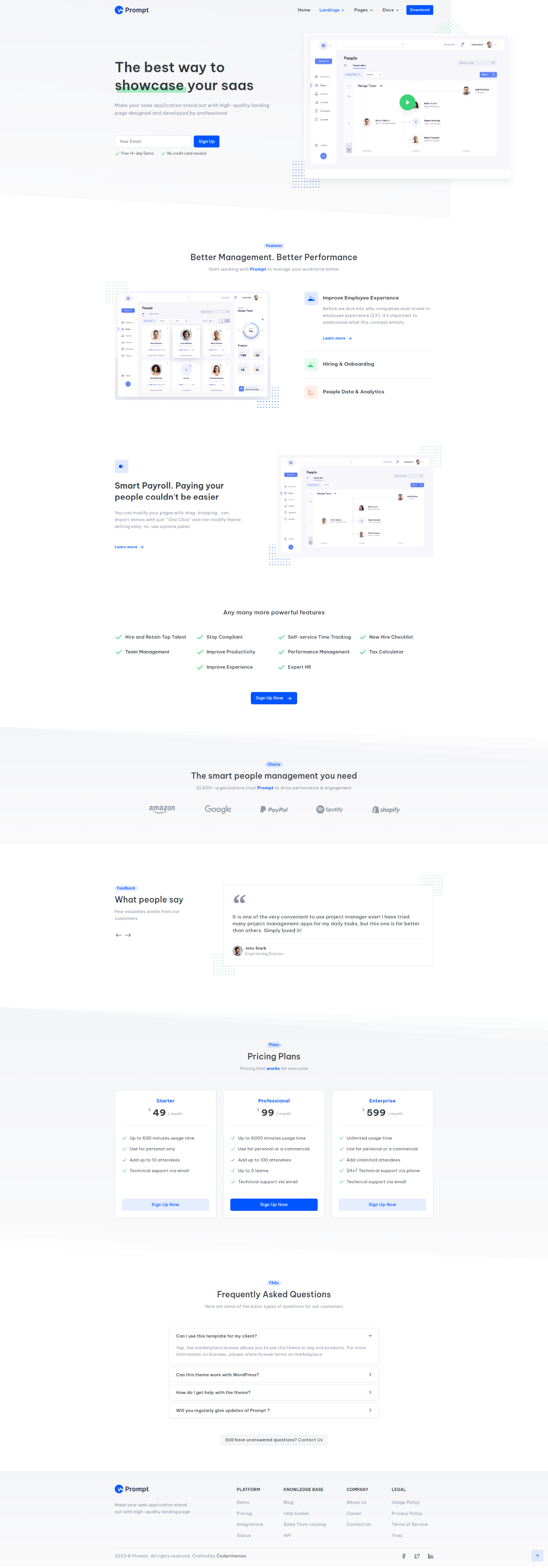This image appears to be a screenshot of a smartphone screen, likely representing a user interface or an app layout. At the very top, there is a grey rectangular banner with black text that reads, "The best way to showcase your [unreadable text]." In the top right corner, there are two small rectangles stacked on top of each other, both outlined in grey with white interiors, though the text inside them is too small to discern. 

Below this top section is another rectangular element that seems to contain five small icons or photos of little people, followed by another icon on the left side. Below these icons, there is a paragraph containing black and blue text, but the text is too small to read clearly.

To the right of this paragraph, there are two more rectangular elements stacked on top of each other, followed by additional black text and a dark blue button. Again, the print is too small to be legible.

Further down, there is a series of rectangles and squares with varying background colors and black text. The first grey rectangle contains black writing, followed by a white rectangle also containing black text. Below this, there is another grey rectangle featuring three squares, each with illegible wording in the middle. The first of these squares has a light blue button beneath it, the second has a dark blue button, and the third has another light blue button.

Between these sections, there is a white rectangle with black and blue text. Further down, there's another grey rectangle with a mixture of blue and predominantly black writing. The very bottom of the page features a few icons, although they are not clearly visible. Overall, the text throughout the screenshot is extremely small and mostly unreadable, making it challenging to determine the exact content or functionality being described.